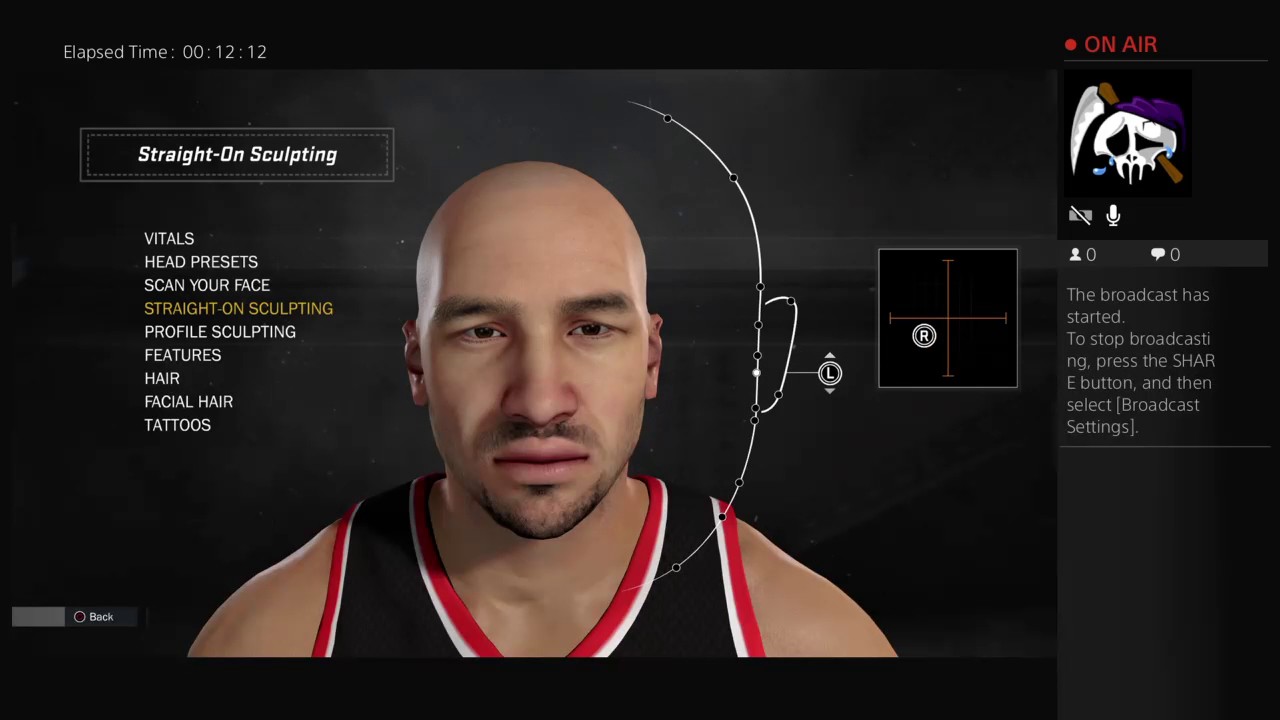This image captures a screen from a character customization interface in a video game. Dominating the scene is the face and upper body of a male character, who has some facial hair and is dressed in a black, white, and red basketball jersey. The background is predominantly black, accentuating the elements on the page.

At the top of the screen, "Elapsed Time: 00:12:12" is prominently displayed, accompanied by a vibrant red "On Air" sign indicating live broadcasting. Adjacent to the sign is a unique emoji: a skull impaled by a sharp axe, adorned with a purple hat. This is followed by a microphone icon and a small avatar icon labeled with the number "0." Similarly, a message icon also shows "0" messages.

A notification reads, "The broadcast has started. To stop broadcasting, press the share button, and then select broadcast settings."

Central to the page is the title "Straight On Sculpting," suggesting a focus on frontal editing of the character’s appearance. Below this title is an extensive list of modification options: vitals, head presets, scan your face, straight on sculpting, profile sculpting, features, hair, facial hair, and tattoos.

The majority of the page is dedicated to displaying the face of the character, framed by an outline, guiding the user through the customization process. The meticulous layout and diverse array of options indicate a sophisticated character customization tool, characteristic of modern video games.